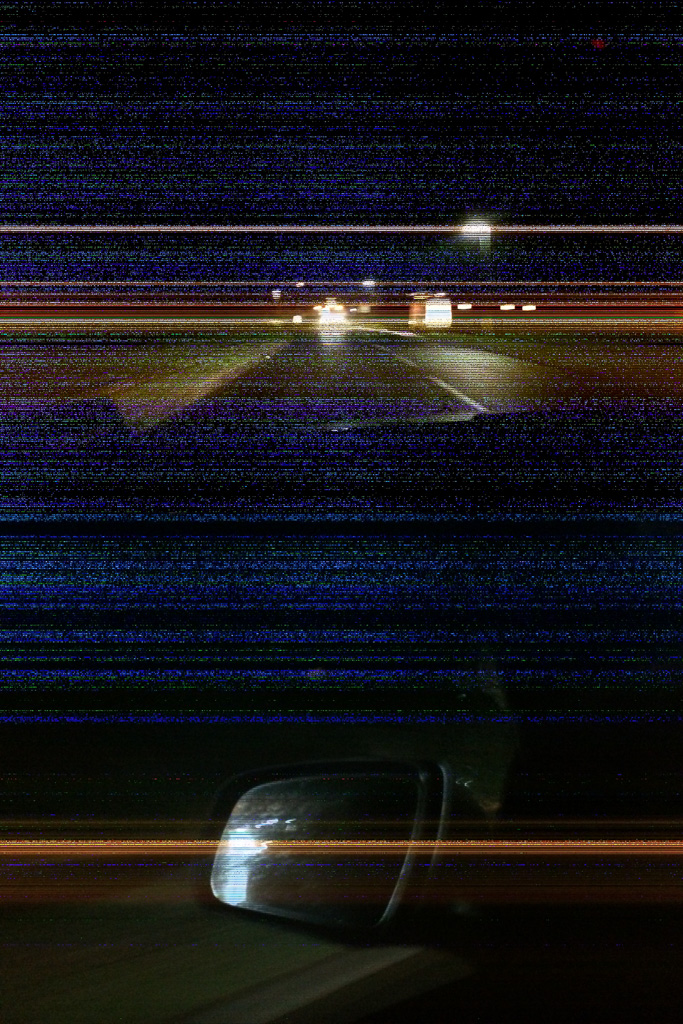The image is of very poor quality, with a significant amount of blur and static lines throughout. The static lines, some in orange and dark blue, are especially prominent across the bottom of the image. Amidst the distortion, there is a vehicle mirror visible in the bottom-center of the frame, against a largely black background. Above the mirror, a road can be faintly made out, with lights dotting the distance. The middle section of the image also features a series of blue static lines, further obscuring the view. Despite the heavy interference, the scene appears to be outdoors at night.